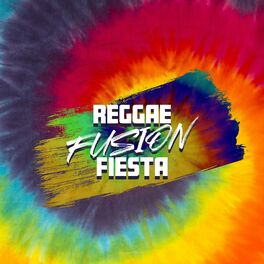The vibrant poster features a mesmerizing tie-dye swirl that radiates from the center in concentric rainbow colors, transitioning smoothly from purple and blue to green, yellow, orange, and red. At the heart of this colorful whirlpool, bold white block letters spell out "Reggae." Beneath that, in a more fluid, cursive-style font, the word "Fusion" gracefully curves, followed by another set of block white letters that conclude with "Fiesta." The overall aesthetic is lively and eye-catching, suggesting a festive event or celebration without providing specific details.